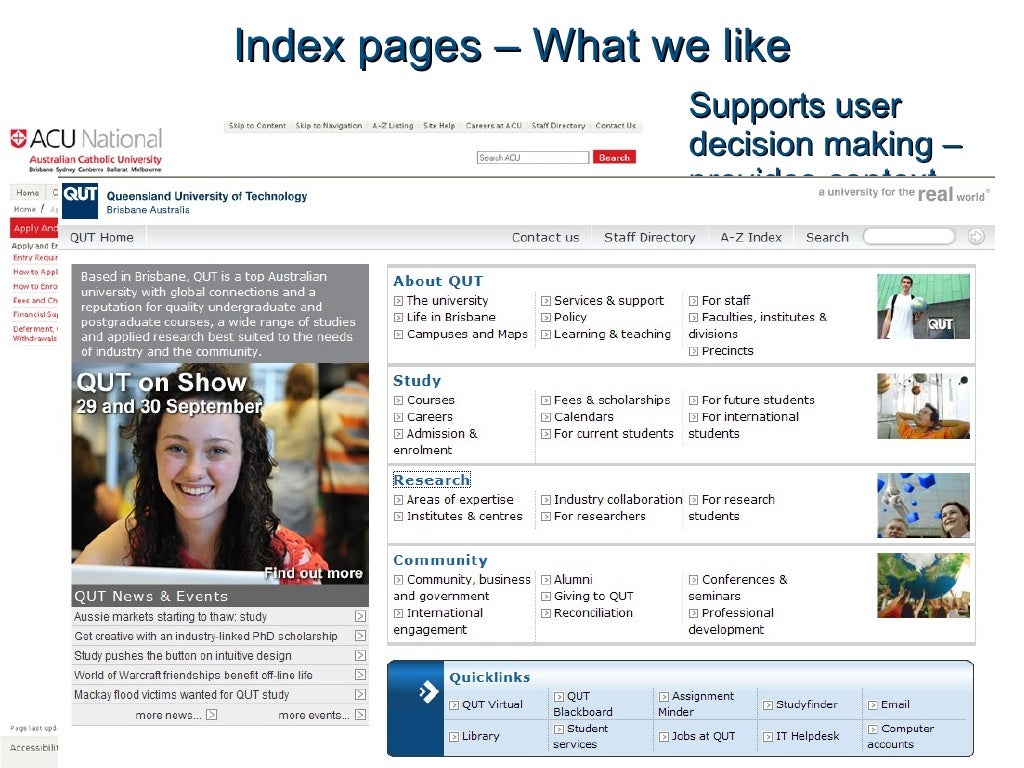The image depicts a webpage with a white background and blue text at the top reading "Index Pages - What We Like Supports User Decision-Making." On the upper left-hand corner of the page, the text "ACU National Australian Catholic University" is visible. Overlaying this main page is another window, also with a white background, bearing the text "Queensland University of Technology, Brisbane, Australia" in the upper left-hand corner.

Prominently featured within the overlaying window is a photo of a smiling university student with long, wavy brown hair. The background shows other students who are blurred out, emphasizing her as the focal point. Surrounding the photo, there is text both above and below it.

To the right of the photo, there is a menu divided into five columns, each with headlines in blue. These headlines read "About QUT," "Study," "Research," "Community," and "Quick Links." The "Quick Links" menu is situated in the lower right-hand corner and distinguished by a blue background.